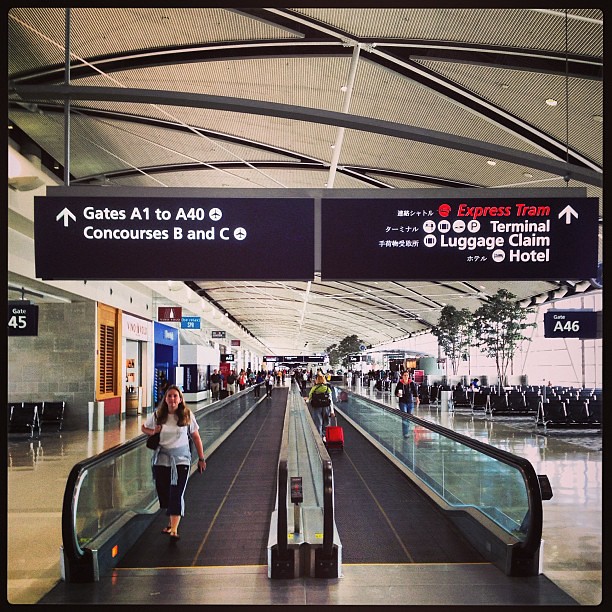The photograph captures a busy airport scene showcasing two black people movers operating in opposite directions under hanging signs. The left-hand sign, in white font on a black background, directs travelers to Gates A1 to A40, Concourses B and C, with an upward arrow and accompanying airplane symbols. The right-hand sign, similarly styled but with "Express Tram" highlighted in red font, indicates the way to the terminal, luggage claim, and hotel, along with some Chinese lettering.

In the foreground, a well-dressed woman with a white shirt, blue sweater tied around her waist, blue striped pants, and black sandals moves toward the viewer on the people mover, carrying a black bag. Another woman heads away on the opposite belt, pulling a red roller bag and wearing a green shirt with blue pants, and carrying a black shoulder bag. There is also a person off the people mover, nearing the camera, identifiable by a blue hoodie with a red interior hood and blue jeans, carrying a white cup of coffee.

The airport’s glossy tan tiles, black waiting seats, and large right-hand windows are prominent features. To the left are some shops, while gate A46's black and white sign stands visible. Overhead, black cables and silver metallic rafters support the hanging signage. Further back, blue and brown signs complement the scene alongside a noteworthy yellow door with a red bottom, and a gray brick wall.